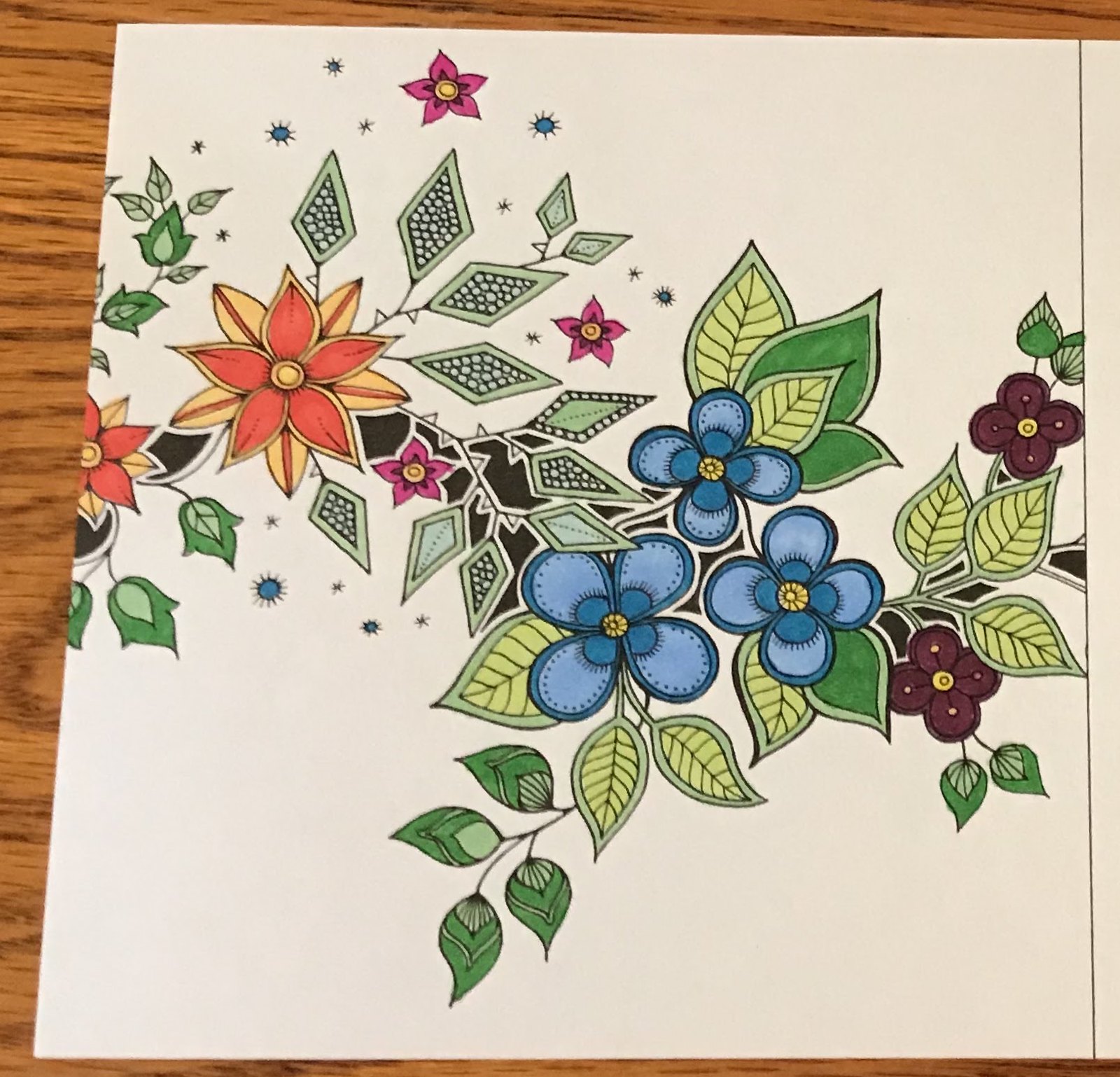A vibrant array of flowers is carefully arranged on a white sheet of paper, which rests atop an orangey-blonde wooden table, showcasing a detailed wood grain pattern. The composition includes green leaves on one side of the image, among which are orange and gold flowers. Scattered around these are additional leaves and white-centered flowers. Prominently featuring are three pink flowers with bright yellow centers, surrounded by some blue, flower-like shapes. The display is further enriched with green leaves adorned with intricate patterns. In another section, dark blue and light blue flowers with yellow centers are visible, accompanied by whiter green and darker green leaves. Adding to the vivid mix are deep plum flowers with yellow centers, framed by light and dark green leaves.